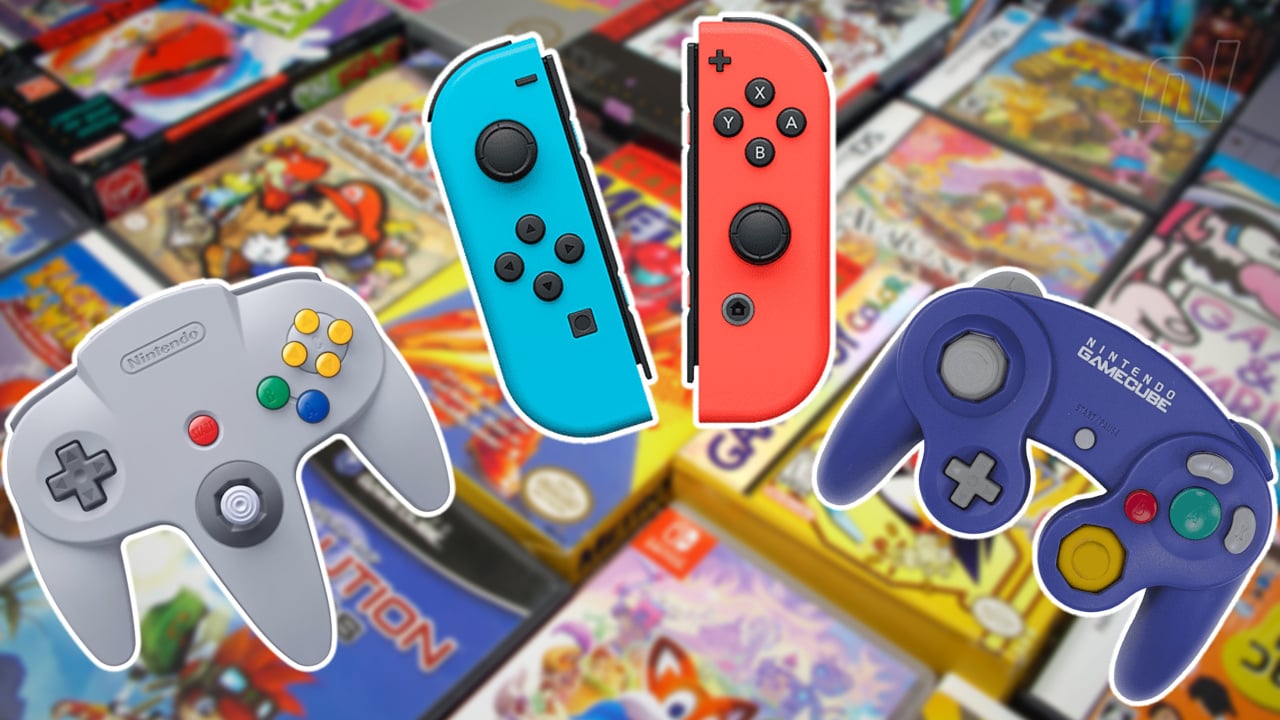The color photograph showcases a collection of three prominent Nintendo game controllers laid out prominently over a display of various Nintendo games. At the center, the iconic red and blue Nintendo Switch Joy-Cons are attached to a mobile game device, featuring a grayscale joystick and traditional gaming buttons. To the left, a gray Nintendo 64 controller stands out with its distinctive three-handle design and colorful buttons in red, green, blue, and yellow. On the right, the classic indigo Nintendo GameCube controller is visible, sporting a similar colorful array of buttons. The controllers rest against a slightly blurry backdrop, depicting an array of Nintendo 64, GameCube, Switch, and DS game cases arranged side-by-side. The image, with its vibrant hues of red, blue, gray, yellow, green, purplish-blue, black, white, and gray, likely represents a promotional setup, possibly for an event or advertisement celebrating Nintendo's gaming legacy.